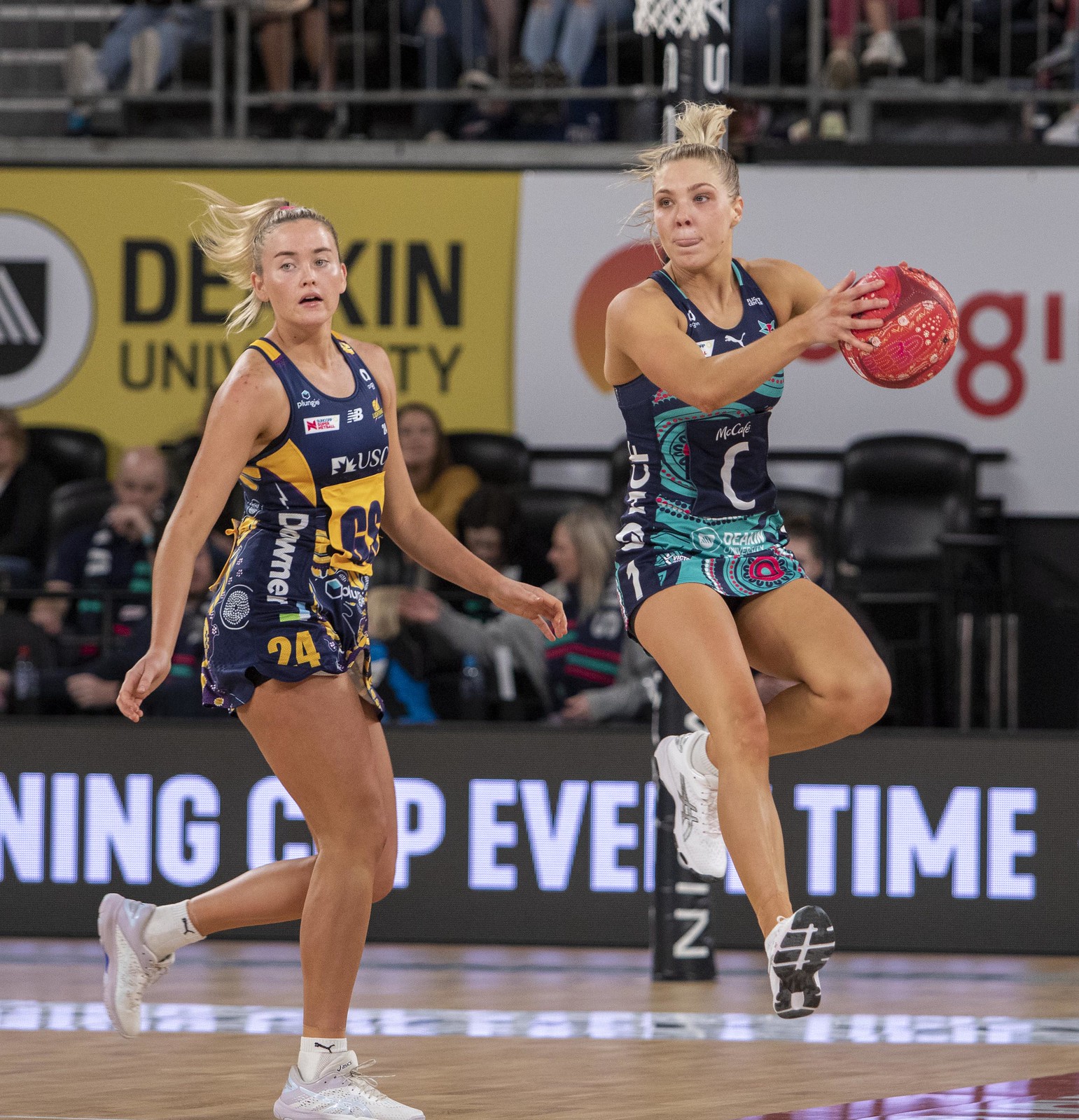In this square image, two women are captured in the midst of an intense volleyball match. The action takes place on a glossy light brown court marked by white and red lines. At the back of the court, a black barrier with white lettering separates the players from a crowd of spectators, who are seated on black chairs in the bleachers. Two large advertisements, one yellow and one white, are positioned above the spectators with a glimpse of a gray gate and more people visible just behind it.

The player on the left is dressed in a blue and yellow uniform with white socks and shoes, her blonde hair tied back in a ponytail, and she faces forward, seemingly ready to defend. The player on the right, also with blonde hair in a ponytail, wears a turquoise and dark blue uniform adorned with sponsorship logos. She is airborne, capturing mid-action as she holds a red and purple volleyball, appearing either poised to throw or having just caught the ball. Her intense focus is highlighted by the detail of her licking her lips, demonstrating the concentration and effort in this moment of professional play.